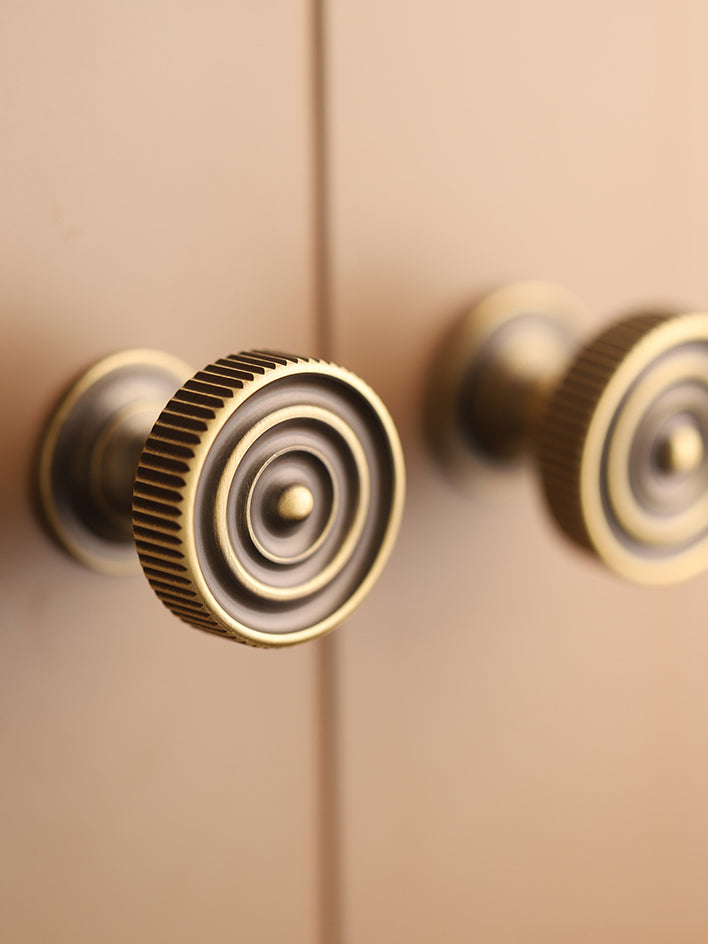The image depicts two cabinet knobs designed to resemble gears, attached to a double-door cabinet with a distinct central line. The cabinet doors are brown with beige shading, and the knobs showcase intricate detailing. Each knob features a central button and a series of concentric circles that create a slightly spiraled effect, transitioning from smaller to larger widths. The outermost edge of the knobs is ridged akin to the edge of a bottle cap, with dark recesses enhancing the texture. The knobs are predominantly brass or bronze in color, with the raised areas catching the light to create a subtle metallic sheen. The knob on the left is sharply focused while the one on the right appears somewhat blurry.